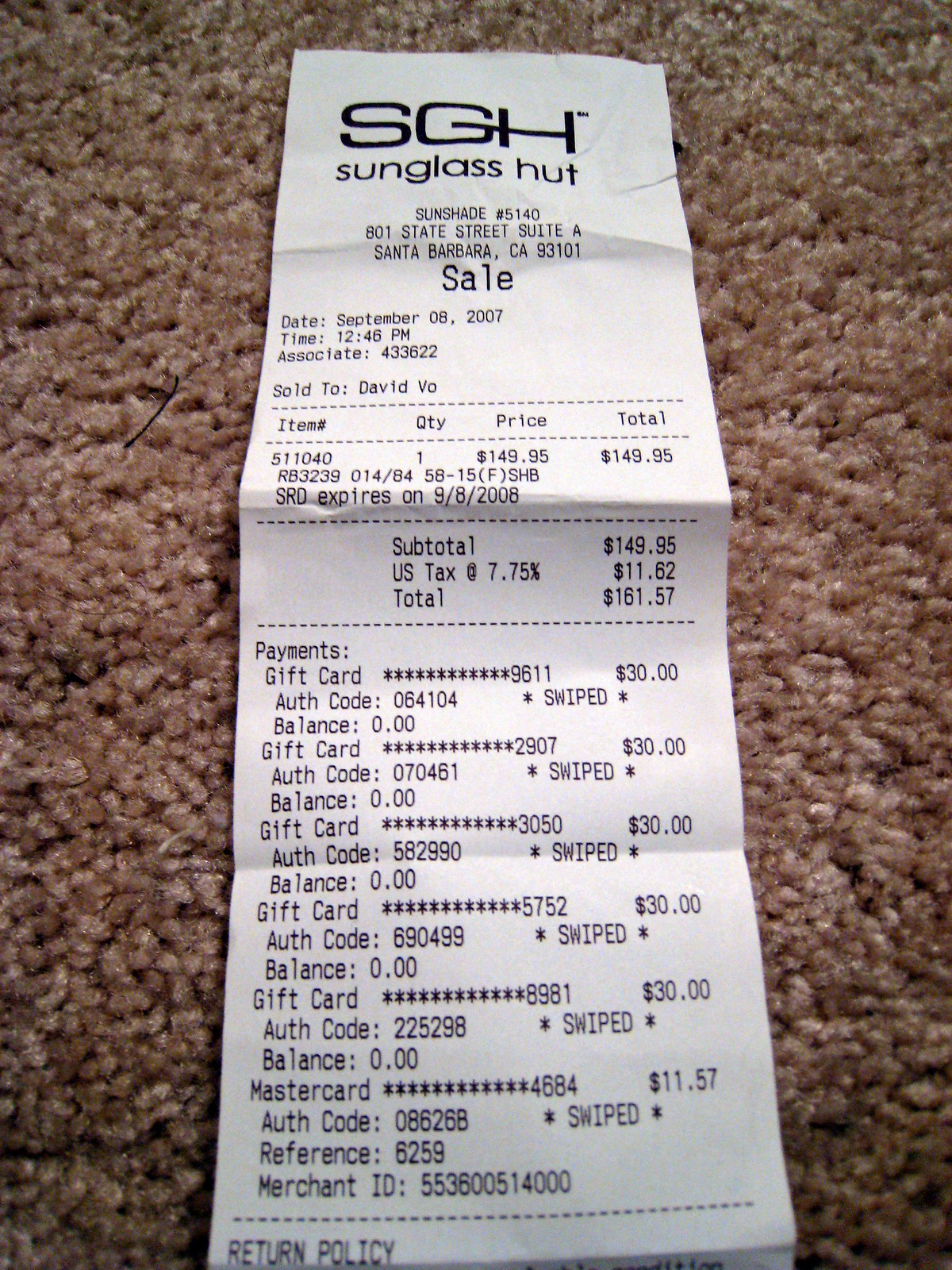A detailed black-and-white receipt from Sunglass Hut, located in Santa Barbara, is laid out on a beige tan carpet. At the top of the receipt, the store's initials "SGH" are clearly printed. Underneath, the recipient’s name, David Vo, is noted, along with the total amount paid, which includes tax, amounting to $161.57. The receipt details that the purchase involved using five gift cards. At the very bottom, the store's return policy is mentioned. Additionally, an associate number, 433622, is printed near the top of the receipt, specifying the employee who handled the transaction. The purchase was made on September 8, 2007, at 12:56 PM.